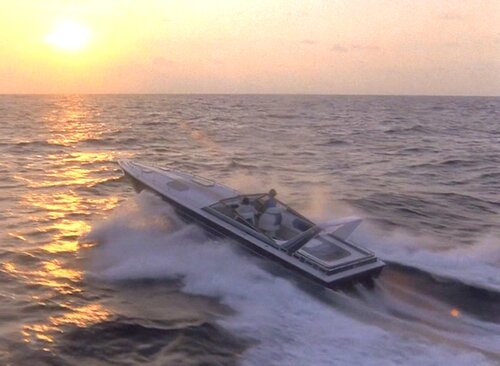In this vivid image, a white speedboat cuts swiftly through the calm ocean waters at sunset, creating a dramatic scene. The boat is clearly traveling at high speed, with jets of water shooting out from behind and frothy white water being pushed away from all sides. The front end of the boat is lifted into the air, suggesting its rapid pace, while the back is partially submerged, stabilized by a high wing near its rear. Inside the open-top speedboat, two passengers are seated on white chairs behind the windshield, one driving while the other enjoys the exhilarating ride. The setting sun casts a golden and orange hue across the sky, reflecting beautifully on the untouched water ahead, enhancing the serene yet thrilling atmosphere of the scene.